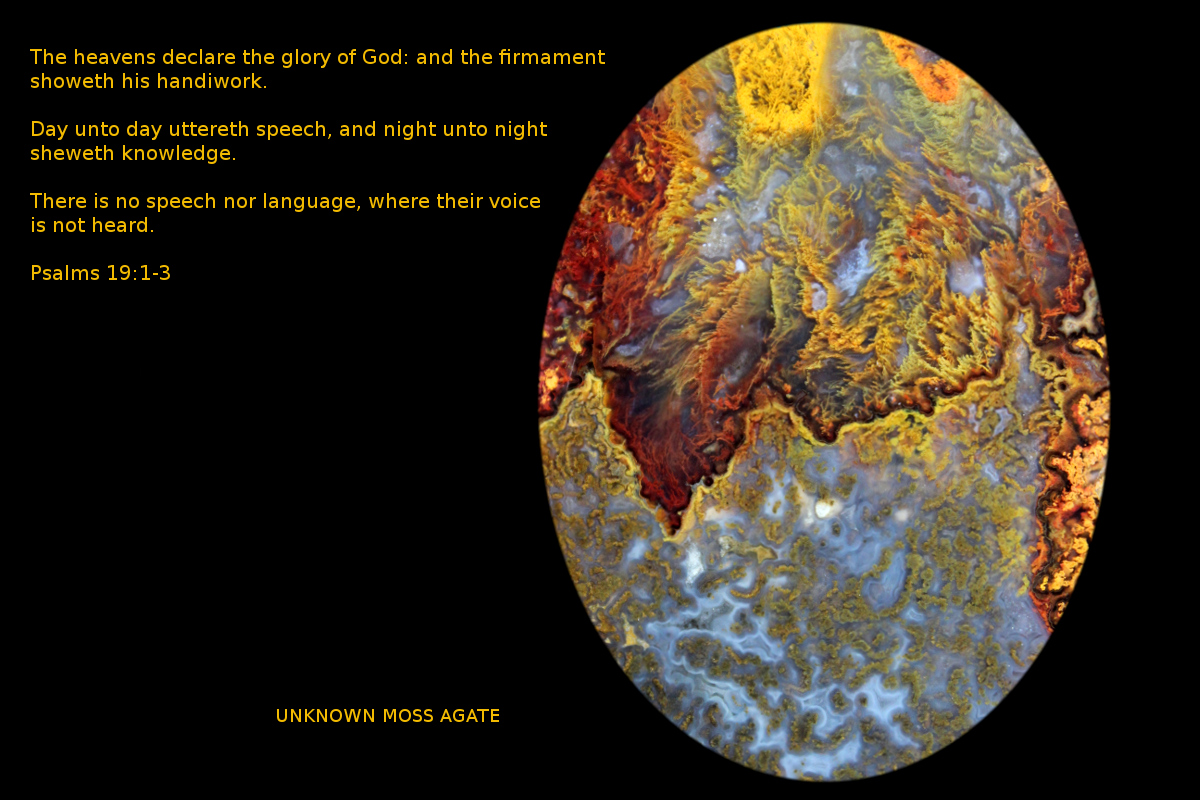The image features a detailed religious diagram, prominently displaying an oval-shaped illustration on the right side, resembling a physical map of the Earth. The map includes intertwined land masses in shades of red, yellow, and brown, surrounded by blue areas that resemble water, all set against a completely black background. On the top left, written in yellow text, are verses: "The heavens declare the glory of God: and the firmament showeth his handiwork. Day unto day uttereth speech, and night unto night sheweth knowledge. There is no speech nor language, where their voice is not heard." At the bottom left of the oval, also in yellow text, is the caption "Unknown Moss Agate." The image incorporates a variety of colors including yellow, lighter yellows, orange, red, blues, blacks, white, and gray, contributing to its visually rich representation.